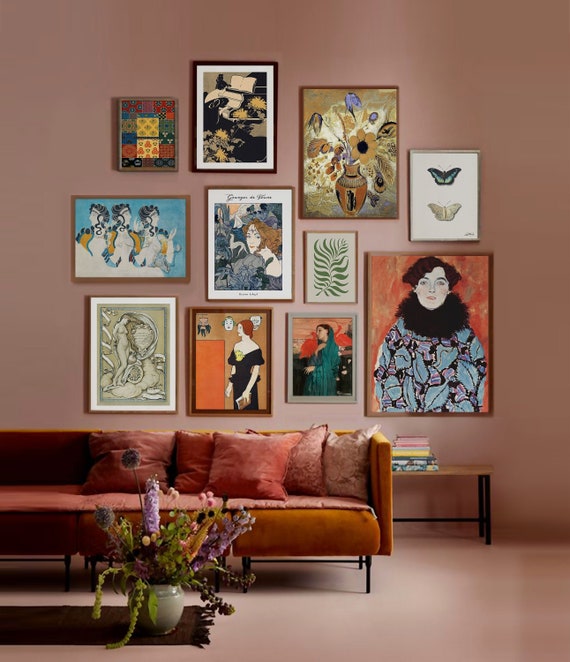This indoor photograph captures a visually engaging room with a cohesive dusky pink color scheme, stretching across both the wall and the flat texture of the floor. The wall is adorned with an eclectic collection of 11 framed paintings of various sizes and techniques, arranged haphazardly and encompassing themes from portraits of women to nature scenes, including butterflies and leaves. Dominating the artwork is a prominent painting of a lady wearing a blue and black top with a black furry collar and short curly brown hair. Below the art display, a plush reddish-orange gradient couch is situated, embellished with five cushions that incorporate shades of pink. In front of the couch, a large gray vase brimming with tall, purple-pink flowers and leaves spilling over its sides is positioned on a thin brown rug with fringed edges. This setting is complemented by a small wooden stand on the right, holding a few books, adding a casual yet refined touch to the space.